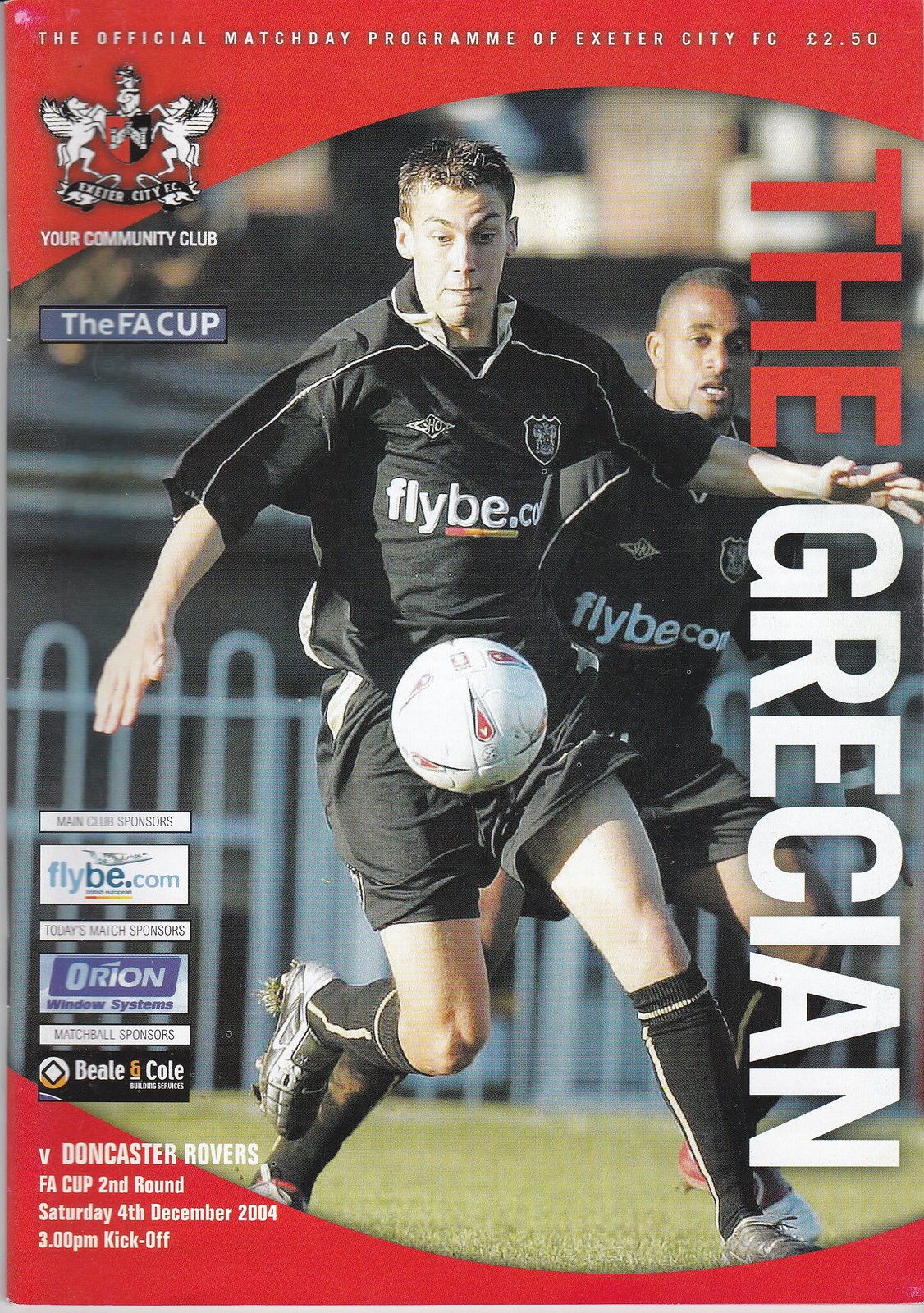This vibrant cover of the official match day program for Exeter City FC features two soccer players engaged in an action-packed moment. Both athletes, clad in black short-sleeved v-neck shirts, shorts, and knee-high socks, are captured mid-play, with the soccer ball positioned near the front player's midsection. The man in the foreground, a white player likely in his 40s, is intensely focused, while a black player in his 30s follows closely behind. The background is slightly blurred, showcasing grassy fields, a fence, and distant buildings.

The top of the cover boasts a bold red arch background with white text reading "The official match day program of Exeter City FC, two pounds 50," alongside a red, black, and white crest. Directly beneath this headline is a smaller inscription, "Your community club." Vertical text along the right side spells out "The Grecian."

At the bottom of the cover, another red arch mirrors the top. In the bottom left corner, white text details the match specifics: "V Doncaster Rovers FA Cup 2nd Round, Saturday 4th December 2004, 3 p.m. kickoff." Accompanied by a series of logos, the sponsors listed include main club sponsors Flybe.com, and match sponsors Orion Window Systems, and Beal and Cole.